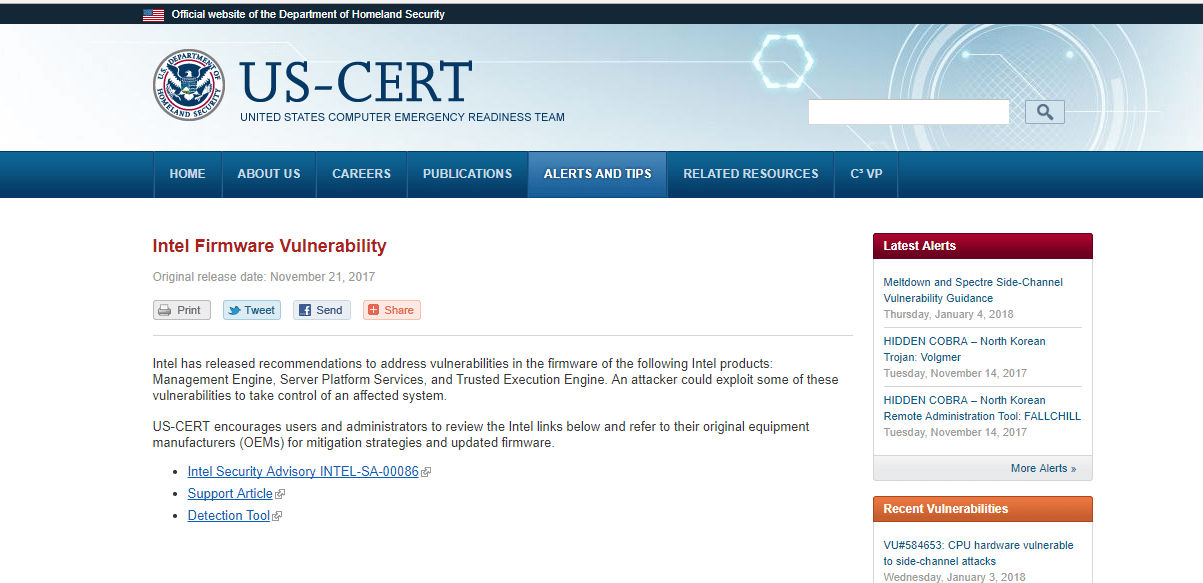The image showcases the homepage of the United States Computer Emergency Readiness Team (US-CERT), a division of the Department of Homeland Security. At the very top, a black banner features a small United States flag icon, accompanied by the text "Official website of the Department of Homeland Security."

Beneath this, a prominent blue section houses the US-CERT's circular logo in blue, red, and white. Adjacent to the logo, the organization's name is displayed in bold blue letters: "United States Computer Emergency Readiness Team." To the right of this text, there is a white search box accompanied by a blue search button marked with a magnifying glass icon.

Following this, a horizontal blue navigation bar presents clickable options: Home, About Us, Careers, Publications, Alerts and Tips (highlighted in a brighter blue), Related Resources, and CVP. The highlighted "Alerts and Tips" tab indicates the section currently being viewed.

Below this navigation bar, a critical update is featured in red text, reading "Intel Firmware Vulnerability," with the original release date noted as November 21, 2017. A series of interactive buttons—Print, Tweet, Send, and Share—are available for user engagement, accompanied by a detailed description.

To the right, a grey box with a red header labeled "Latest Alerts" lists recent alerts, providing a link to view more. Beneath this, another grey box with an orange header titled "Recent Vulnerabilities" lists the latest identified threats.

Overall, the website's structured layout prioritizes accessibility and comprehensive information dissemination related to cybersecurity alerts and vulnerabilities.